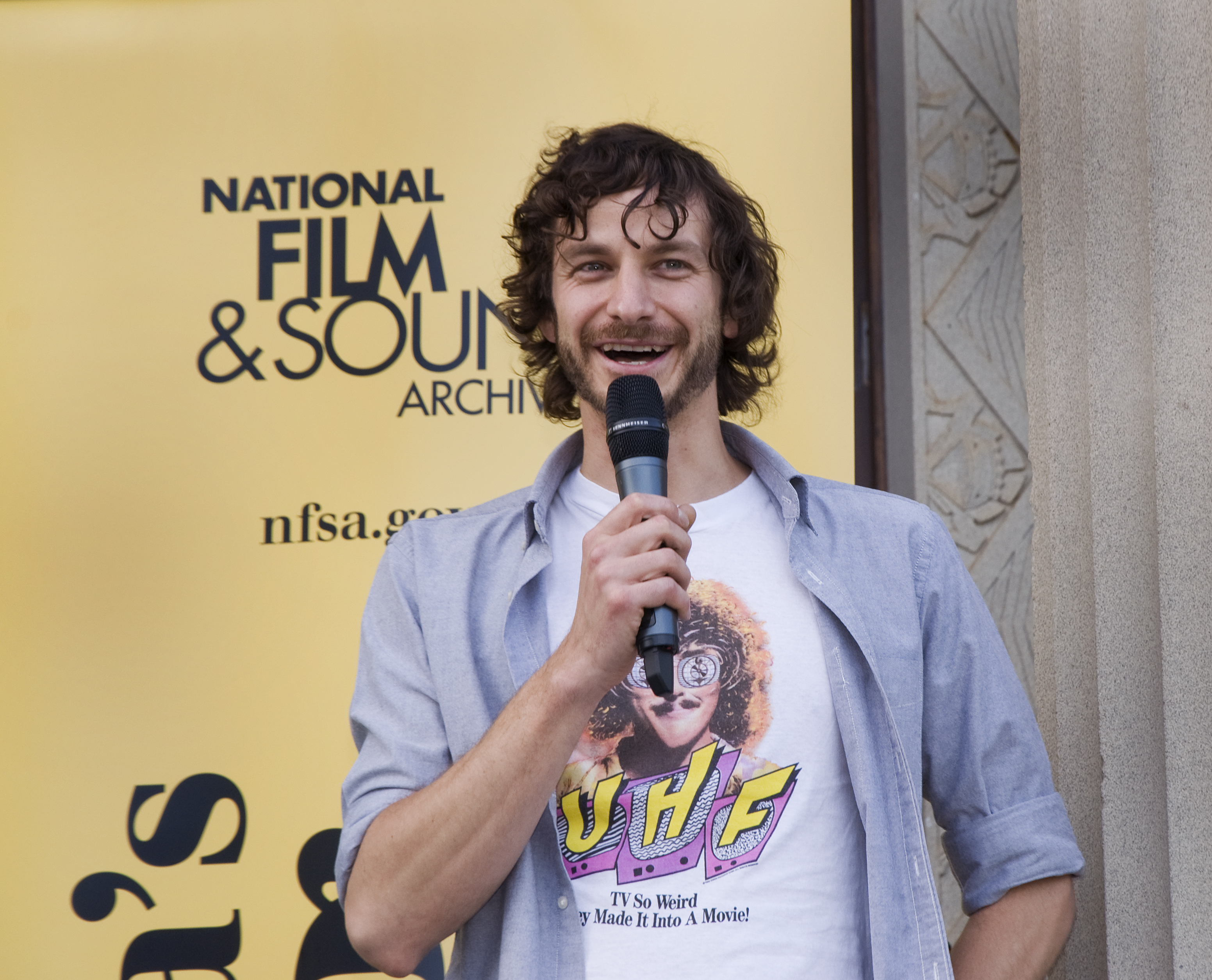The image features Dean Lewis standing in front of a yellow banner that reads "National Film and Sound Archive, NFSA.gov." He is holding a black microphone in his right hand and appears to be speaking, as his mouth is open in a smile. Dean is dressed in a white t-shirt with the text "UHF" in white lettering amidst drawings of TVs with static backgrounds, and the phrase "TV so weird they made it into a movie" in black text below. Over this, he wears an open blue button-up shirt with the sleeves rolled up. He has short curly brown hair, and brown facial hair that frames his cheeks, jaw, and upper lip. There is a concrete pillar partially visible to his right, creating a contrast against the otherwise vibrant backdrop.